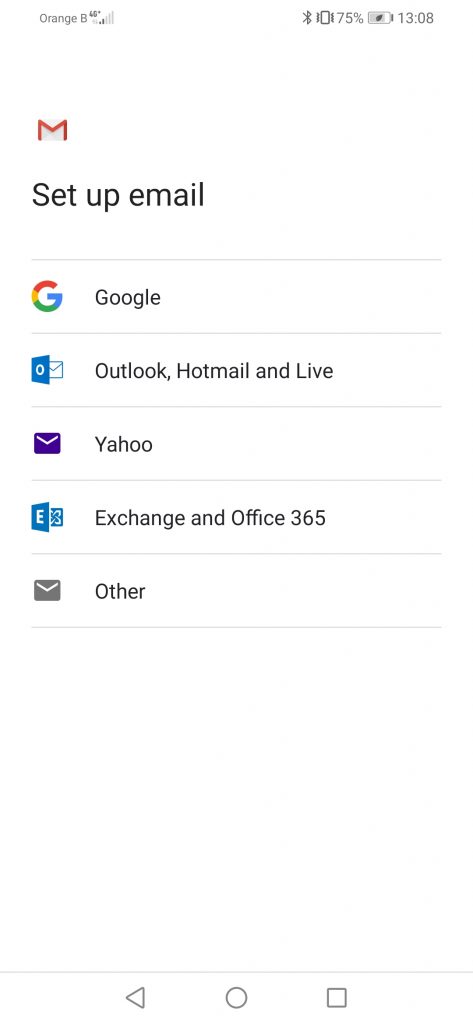The image is a screenshot of a smartphone display with a predominately white background. 

At the very top, in a small gray font, the word "Charge" can be seen, indicating the phone's charging status. The top bar also displays the current weather at 66 degrees, although it's unclear whether this is in Fahrenheit or Celsius. Additionally, there is a Bluetooth icon and a battery life indicator showing 75%. The time is shown in military format as 13:08, which converts to 1:08 PM in standard time.

Just below the top bar, slightly to the left, the Gmail logo is visible. The logo is a thin red 'M'. Below this, in a larger black font, the text "Set up email" is prominently displayed.

Following this title, there are five options for setting up different email accounts, each separated by thin gray lines:
1. Google
2. Outlook, Hotmail, and Live
3. Yahoo
4. Exchange and Office 365
5. Other

To the left of each option, corresponding logos are displayed:
- Google’s logo is a multicolored 'G' in red, yellow, and blue.
- Outlook's logo resembles a blue letter or computer screen.
- Yahoo’s logo is a purple envelope.
- Exchange and Office 365 share a similar logo featuring an 'E' and an 'O'.
- The "Other" option uses a gray envelope icon, depicting the backside of an envelope.

The clean layout and clear options indicate a user-friendly interface for setting up various email accounts on the smartphone.